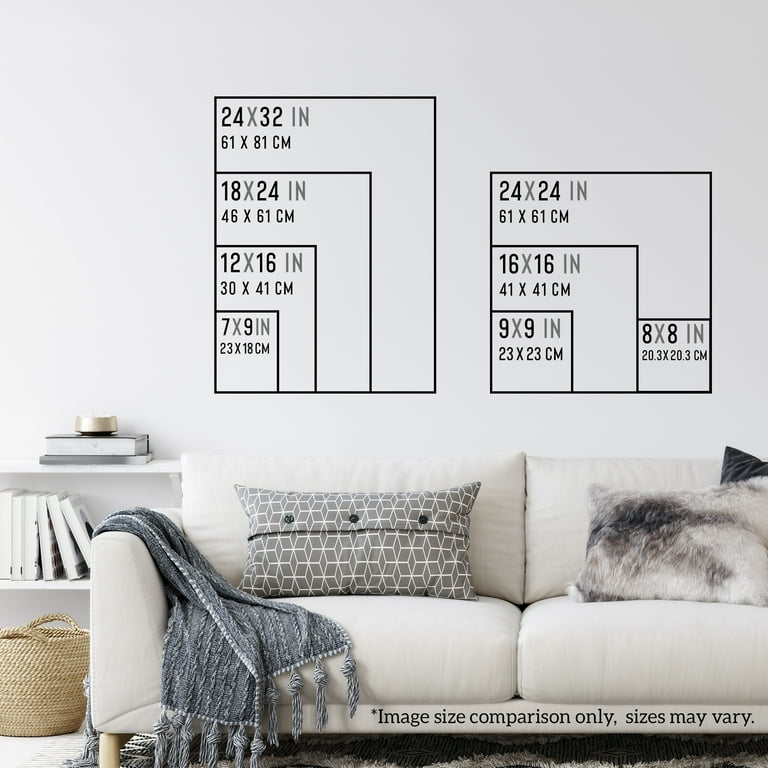The image showcases a white sofa adorned with two distinct throw pillows: one is fur-like with a combination of white and brown colors, while the other is white with a gray design and features three buttons. A small gray throw blanket is casually draped over the sofa. Positioned against a light gray wall, the scene includes white shelves nearby, home to a few books and a candle. Below the shelves, a brown wicker basket rests on the floor. The wall behind the sofa is decorated with diagrammatic measurement blocks, showing various frame sizes, such as 24 by 32 inches (61 by 81 cm), 18 by 24 inches (45 by 61 cm), 12 by 16 inches (30 by 41 cm), and 7 by 9 inches (18 by 23 cm), among others. These blocks serve as visual guides for image or item sizing with a note in black font reading, "Image size comparison only, sizes may vary." Beneath the sofa lies a simple rug, completing the minimalist and informative display, likely intended for a furniture advertisement.